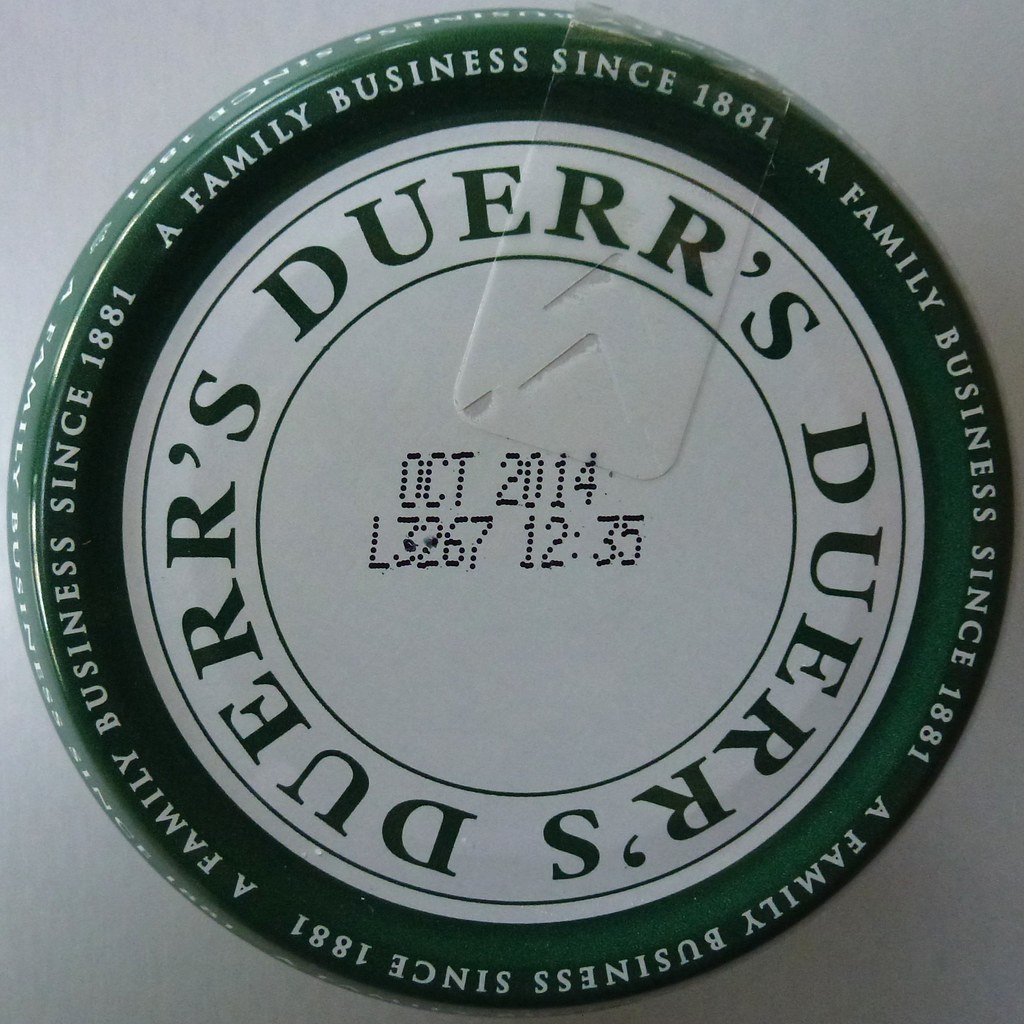The image features a bottle cap prominently in the center, showcasing a simple yet detailed design. The cap is primarily white with dark green lettering and has a dark green rim around it. At the top of the cap, in white text on a green background, it reads, "A family business since 1881," encircling the perimeter. Within this outer text, there is a bold inscription that says "DUEERR'S" (stylized as D U E R R apostrophe S) in dark green letters on a white background. Also stamped on the cap is the date "October 2014," indicating when it was made. The cap resembles those found on soda or Snapple bottles, though only the cap is visible in the image. The overall setting is simple, as the bottle cap appears to be placed on a table.